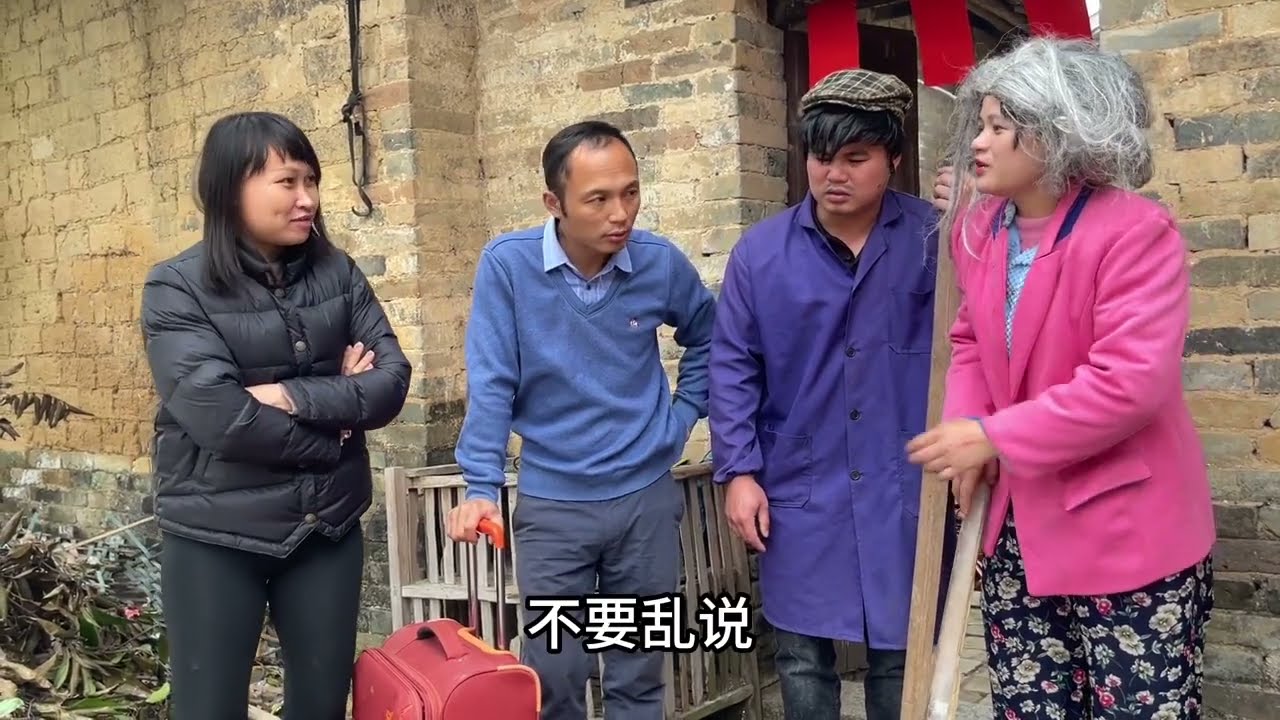The photograph depicts an Asian family of four standing outdoors in front of a light brown brick wall with a doorway to the right adorned with three red fabric flags. The family, dressed in warm clothing indicating a cold day, appears to be preparing for a trip but is momentarily delayed. 

On the left is a woman with black hair, wearing a down ski jacket and black pants, with her arms folded. Next to her is a man with dark hair, slightly balding, dressed in a blue v-neck sweater over a collared shirt and gray pants. He is leaning on the handle of a red upright suitcase. 

To his right, a man in a plaid flat cap, wearing a long purple coat and blue jeans, is holding an object that might be a walking stick. The last person on the far right is a woman with gray, possibly wigged hair, clad in a pink blazer, a blue top, and floral print pants.

The mother seems to be talking to the family, and despite standing outside the doorway, they all seem attentive and engaged, suggesting a significant moment before their departure. The scene carries an air of comedy or theatricality, possibly indicating this is a staged or scripted scene. Additionally, the presence of undeciphered Asian language text in the middle of the picture hints at a cultural or narrative context that is specific to their background.